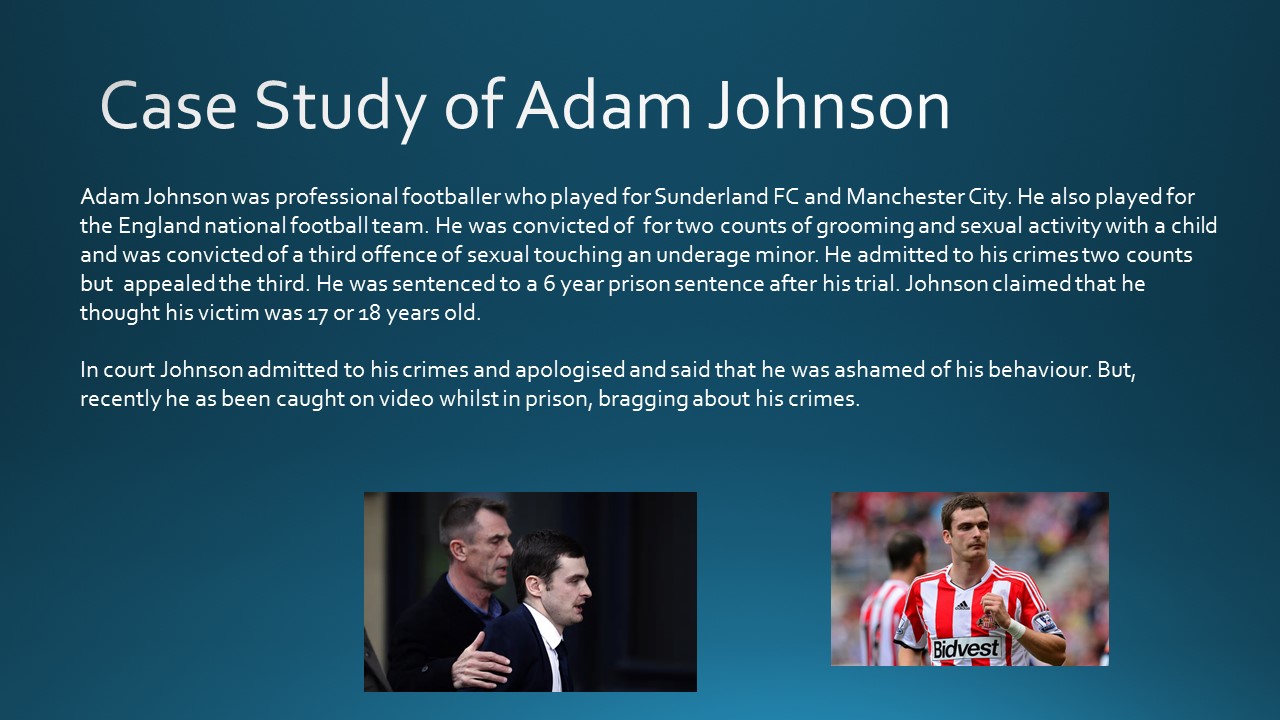On a dark silver-blue background with stark white lettering, this image features two small photos at the bottom and the headline "Case Study of Adam Johnson." The left photo shows two well-dressed men, both with black hair, walking side by side; the taller man has his arm on the other man's shoulder. The right photo depicts Adam Johnson in a white jersey with red vertical stripes, emblazoned with "Bidvest," playing football with another player seen looking away behind him. 

The text narrates the story of Adam Johnson, a professional footballer who played for Sunderland FC, Manchester City, and the England national football team. He was convicted of two counts of grooming and sexual activity with a child and a third offense of sexually touching an underage minor. Despite admitting to and apologizing for two of his crimes, claiming he believed the victim to be 17 or 18 years old, Johnson appealed the third count but was ultimately sentenced to a six-year prison term. Recently, Johnson was filmed in prison boasting about his crimes, contradicting his earlier expressions of shame.